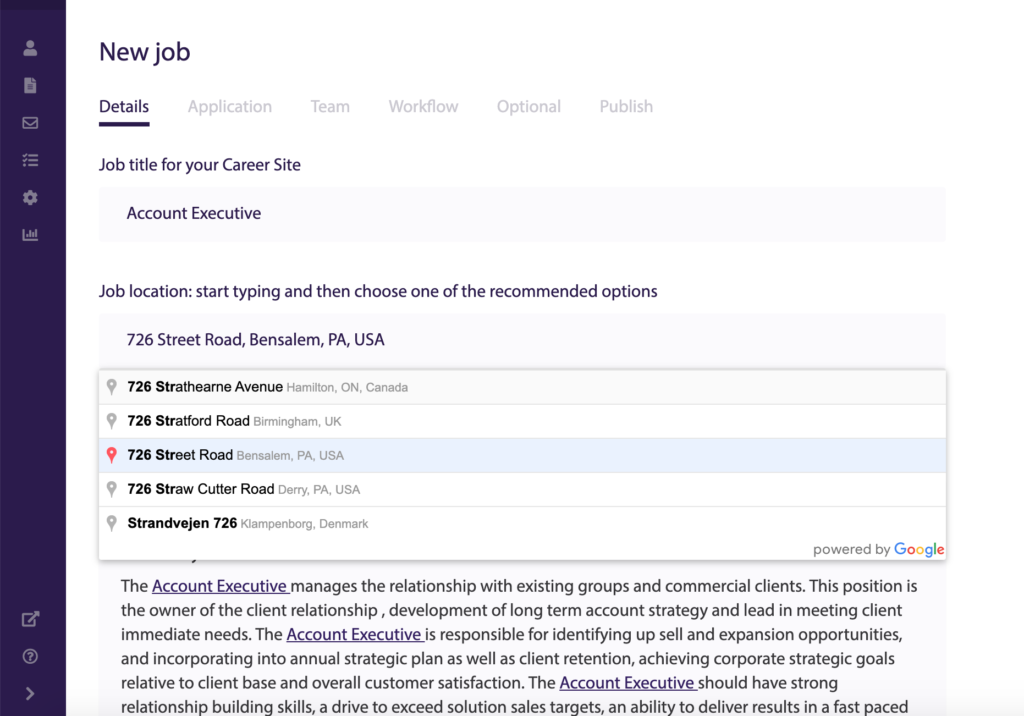The image showcases a user interface for posting a new job. At the top of the page, there is a prominent title that reads "New Job." Below the title, several sections are listed: Details, Application, Team, Workflow, Optional, and Publish.

The "Details" section is currently in focus. Here, the job title is specified as "Account Executive." The section following instructs the user to type the job location and then select one from a list of recommended options. An example address, "726 Street Road, Bensalem, PA, USA," is shown, along with other similar location suggestions.

Underneath, the "Description" area provides an overview of the Account Executive role:

"The account executive manages the relationship with existing groups and commercial clients. This position is the owner of the client relationship, development of long-term account strategy, and lead in meeting client immediate needs. The account executive is responsible for identifying upsell and expansion opportunities and incorporating them into an annual strategic plan, as well as client retention. Achieving corporate strategic goals relative to the client base and overall customer satisfaction. The account executive should have strong relationship-building skills, a drive to exceed solution sales targets, and an ability to deliver results in a fast-paced environment."

The remainder of the job description is cut off.

On the left side of the interface, there is a navigation pane in a navy-purple color, which contains eight icons. The top section of the pane features five icons, and the bottom section has three more. The overall design of the page is clean and minimalistic, predominantly featuring white and black text with accents of light purple.